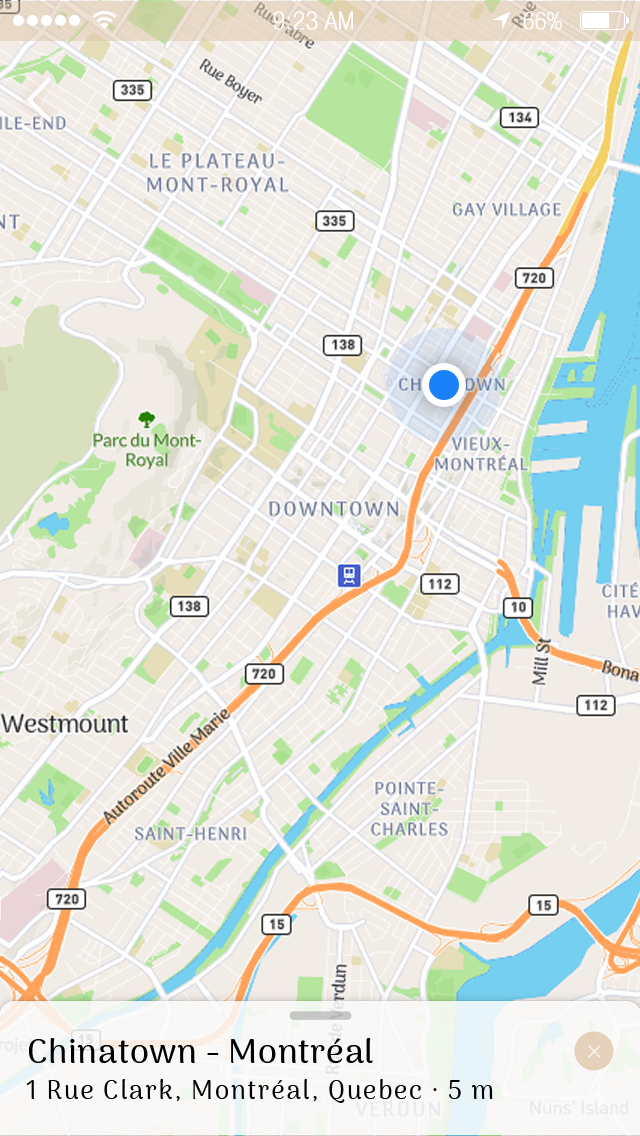A vibrant, color graphic showcasing the interface of a street navigation app on a smartphone. At the top, a transparent rectangular bar displays the standard smartphone icons: the time, shown as 9:23 AM in white text, and a battery icon indicating 66% charge, positioned on the right. Below is a slightly transparent white rectangle with the destination "Chinatown-Montréal" prominently displayed, followed by the address "1 Rue Clark, Montréal, Quebec."

Central to the map is a blue dot encircled by a white ring, pinpointing the location over the text "Chinatown." The map features a major road diagonally bisecting the screen from the upper right to the upper left, labeled "720" within a white rectangle with a black border, noting it as Autoroute Ville-Marie. On both sides of the image, street scenes of this Montréal neighborhood are depicted with various diagonal lines, indicating the intricate roadways branching out. Additionally, a water inlet starts at the upper right of the map, cutting across diagonally before exiting at the lower-left edge. This graphic offers a detailed and navigable view of Chinatown in Montréal.